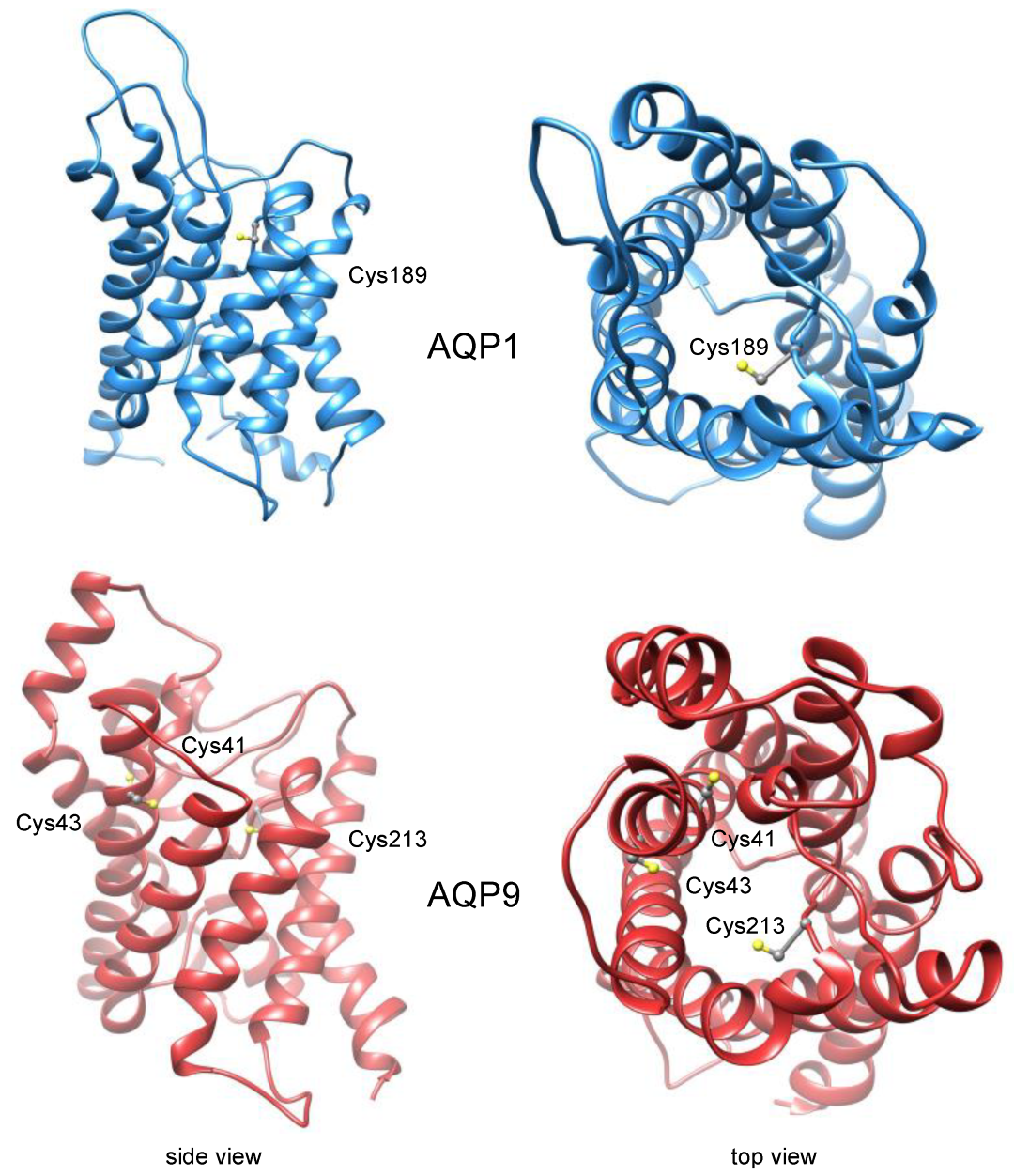The image displays various structures resembling twisted wires or paper, potentially indicating a chemical or molecular composition. In the center, bold capital letters spell out "AQP1," set against a blue background. Two blue images dominate the top section: the left one labeled "CYS189" and the right one "CSY189." These intricately twisted forms appear to highlight specific molecular structures or products.

Below, two red images provide a contrasting view and add further detail. The image on the far left is marked "side view," with labels "CYS213," "CYS41," and "CYS43," showing heavily twisted structures. To the right, another red image labeled "top view" offers a more complex arrangement with curls and twists, accompanied by labels "CYS214," "CYS43," and "CYS41."

Overall, the combination of blue and red images with detailed labels suggests a detailed representation of some chemical or molecular components.